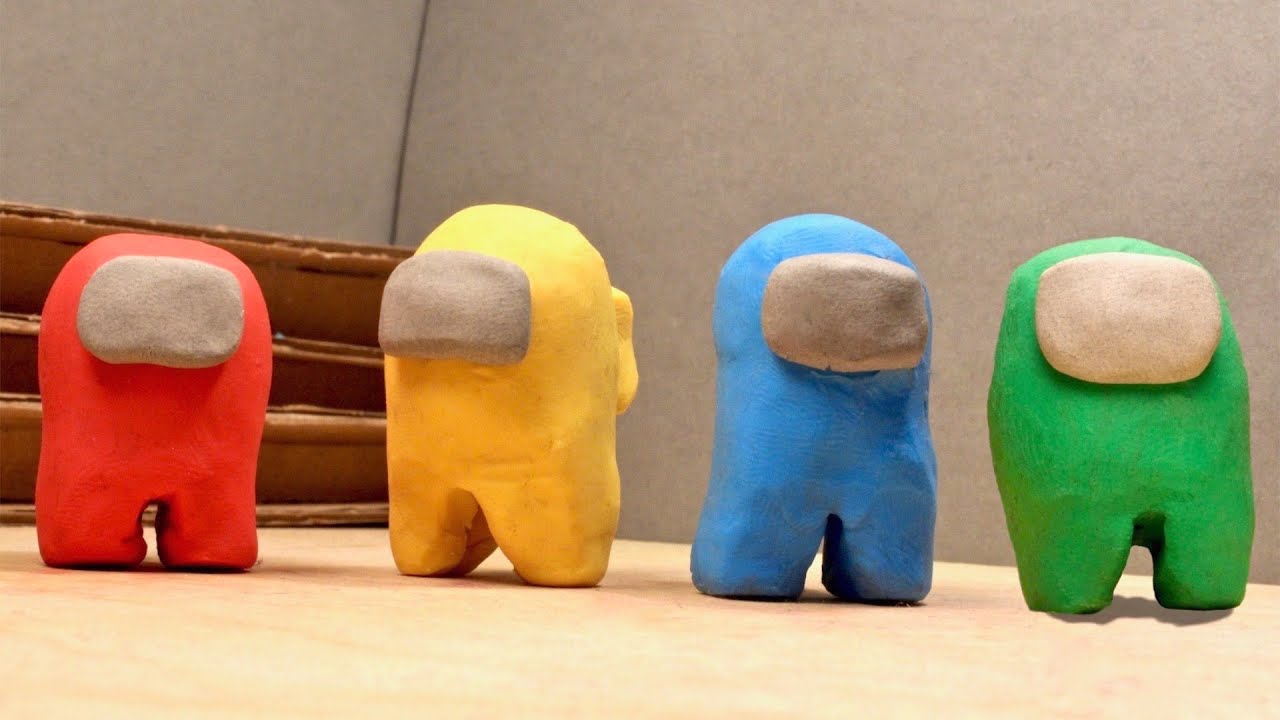This color photograph depicts four simplified humanoid figures meticulously crafted from colored clay, each standing aligned from left to right in a rectangular frame. The scene is set against a backdrop that consists of brown cardboard resembling the side of a box and a darker brown wall, almost taupe in color, providing a muted yet warm ambiance. The figures, which share an overall simplistic design, feature rectangular bodies with rounded tops and rectangular legs, akin to teeth or basic humanoid shapes. Each figure is adorned with a square piece of brown clay where the face would typically be, though no other facial features are present.

From left to right, the four figures are distinctly colored in vibrant hues: red, yellow, blue, and green. They stand on a light brown surface, possibly a table or a desk, with an additional piece of cardboard visible on the left side of the image. The uniformity of their shapes and the minimalistic design gives them a somewhat whimsical appearance, reminiscent of playtime creations made from Play-Doh, evoking a sense of simple, playful artistry.